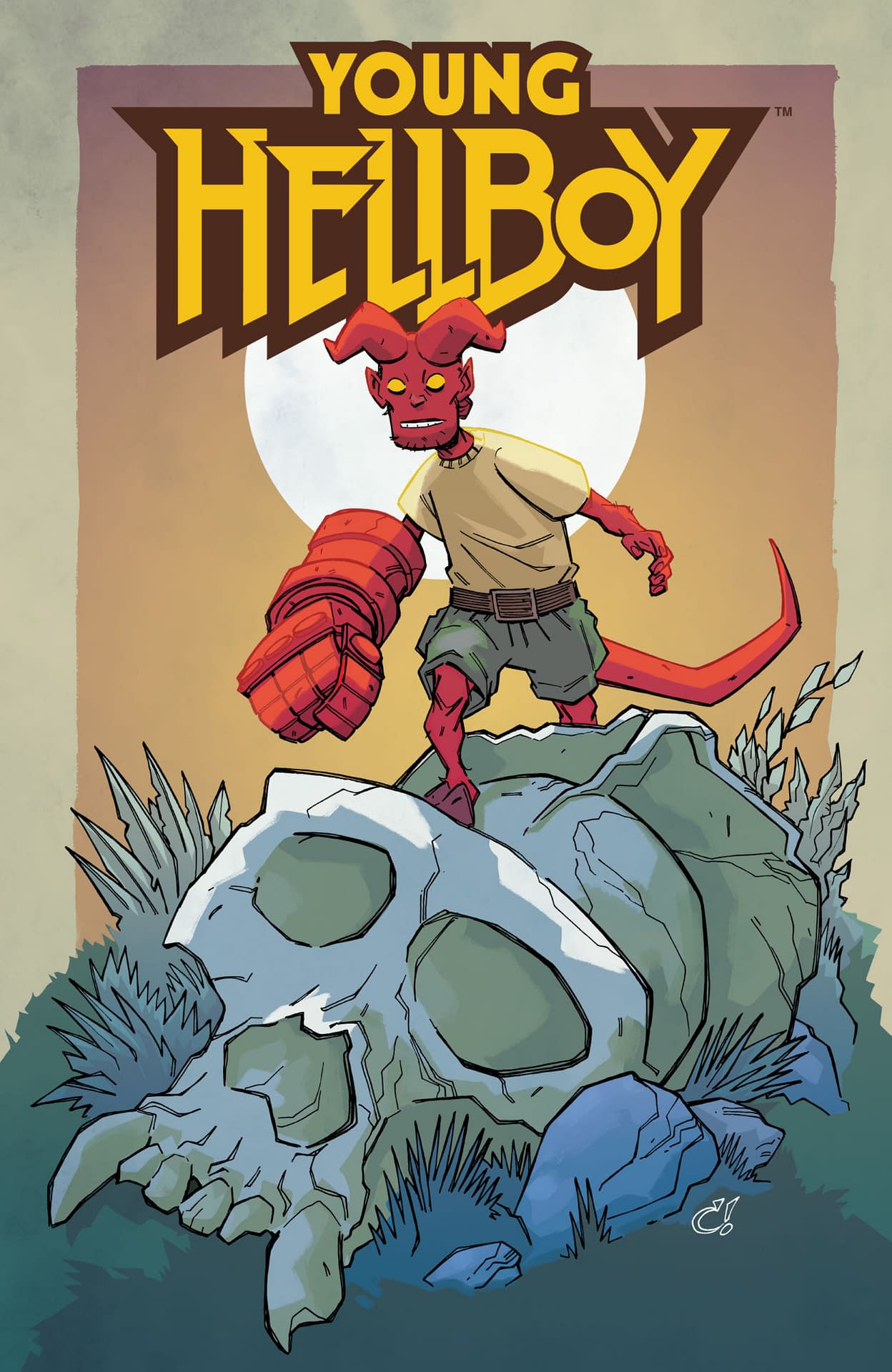This vibrant digital artwork for a comic book cover, titled "Young Hellboy," features a striking scene set in a desaturated, twilight landscape. Dominating the foreground is a very large, tan skull resembling that of a mythical cryptid or giant gorilla, partially obscured by overgrown leaves, brush, and rocks. This imposing skull serves as the climbing ground for Young Hellboy, a red demon-like creature with yellow eyes, a long red tail, large red horns protruding from his head, and one notably large hand. He's depicted wearing a tan shirt and dark gray shorts secured with a brown belt, showcasing a readiness for adventure. The background transitions from purple to yellow, suggesting a late afternoon with the sun setting, adding a dramatic contrast to the scene. A prominent art logo, consisting of a "C" with an exclamation point, is situated towards the bottom right. The top of the image boldly bears the title "Young Hellboy" in large, sharp yellow letters, anchoring the composition. The playful, adventurous vibe is encapsulated in the cartoonish yet detailed portrayal of the character and his surroundings.